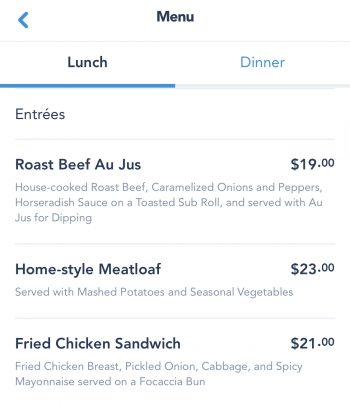The image showcases a detailed close-up of a lunch menu. At the top, "Menu" is prominently displayed, followed by two sections labeled "Lunch" and "Dinner," with "Lunch" being selected. The Entrees section features three offerings:

1. **Roast Beef au Jus ($19)**: This dish includes house-cooked roast beef complemented by caramelized onions and peppers, accompanied by horseradish sauce. The roast beef is served on a toasted sub roll with au jus sauce available for dipping.

2. **Home Style Meatloaf ($23)**: A serving of traditional meatloaf, paired with creamy mashed potatoes and a selection of seasonal vegetables. 

3. **Fried Chicken Sandwich ($21)**: A crispy fried chicken breast topped with pickled onions, cabbage, and a spicy mayonnaise. This entrée is served on a freshly-baked focaccia bun.

Each entree is meticulously described, highlighting both ingredients and accompanying sides, along with their respective prices. This detailed lunch menu offers a range of hearty, comforting dishes.